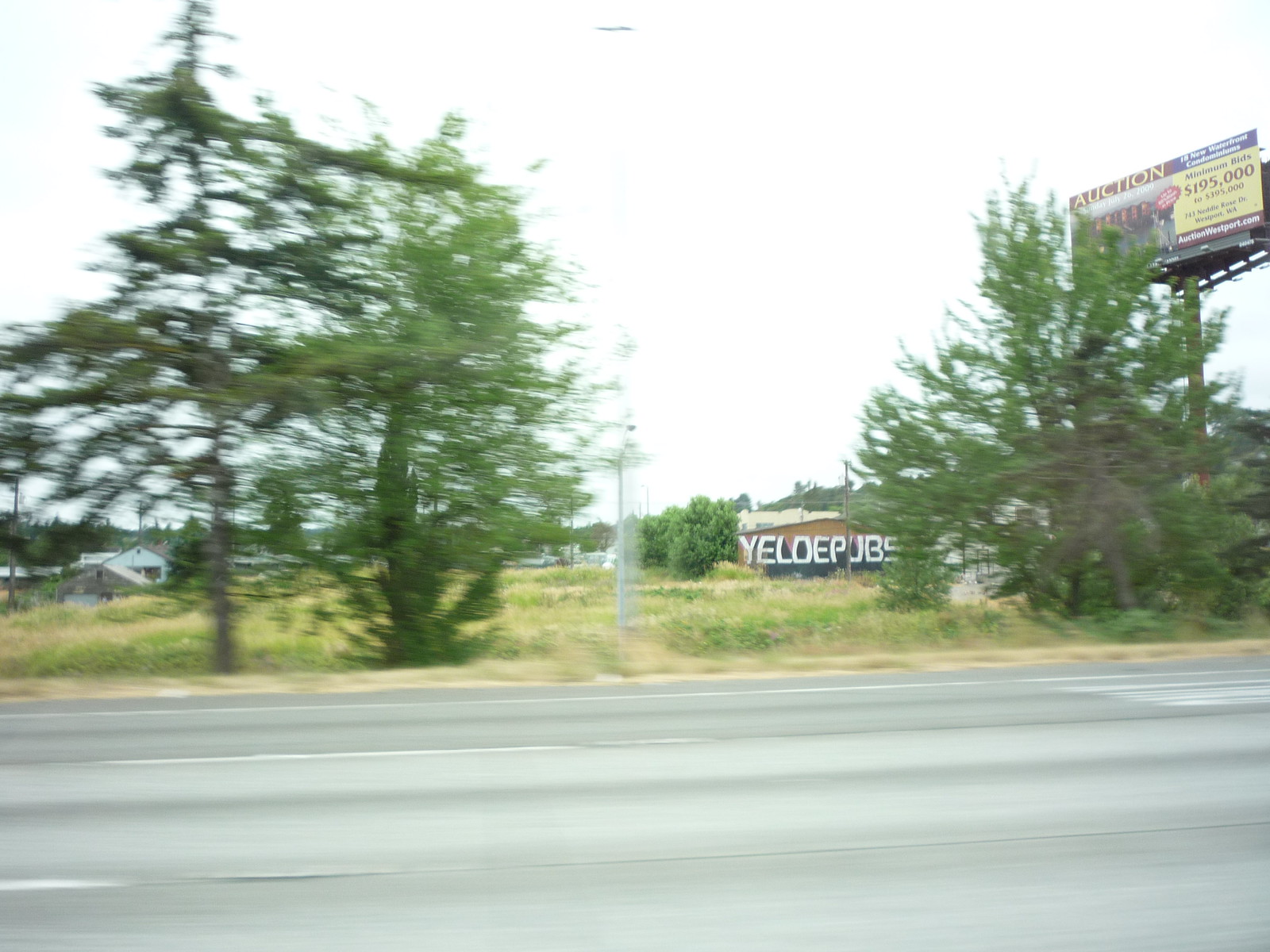A blurry photograph captures a deserted highway with no visible cars. Surrounding the road are lush green trees and patches of grass both near and far. Short grass lines parts of the scene, offering a natural border. In the distance, we can see quaint white houses alongside a few brown or gray houses with pitched roofs, creating a picturesque impression of a small community. Among these structures is a distinct brown building with some writing on its side, reading "Yelo Pubs," although it's unclear if this is graffiti or a faded sign. Further elements in the image include several telephone poles standing along the edge of the highway, adding to the rural ambiance. In the top-right corner, a prominent billboard advertises an auction for "18 new waterfront condominiums" in Westport, Washington, with a range of minimum bids from $195,000 to $395,000 and further details available at AuctionWestport.com.